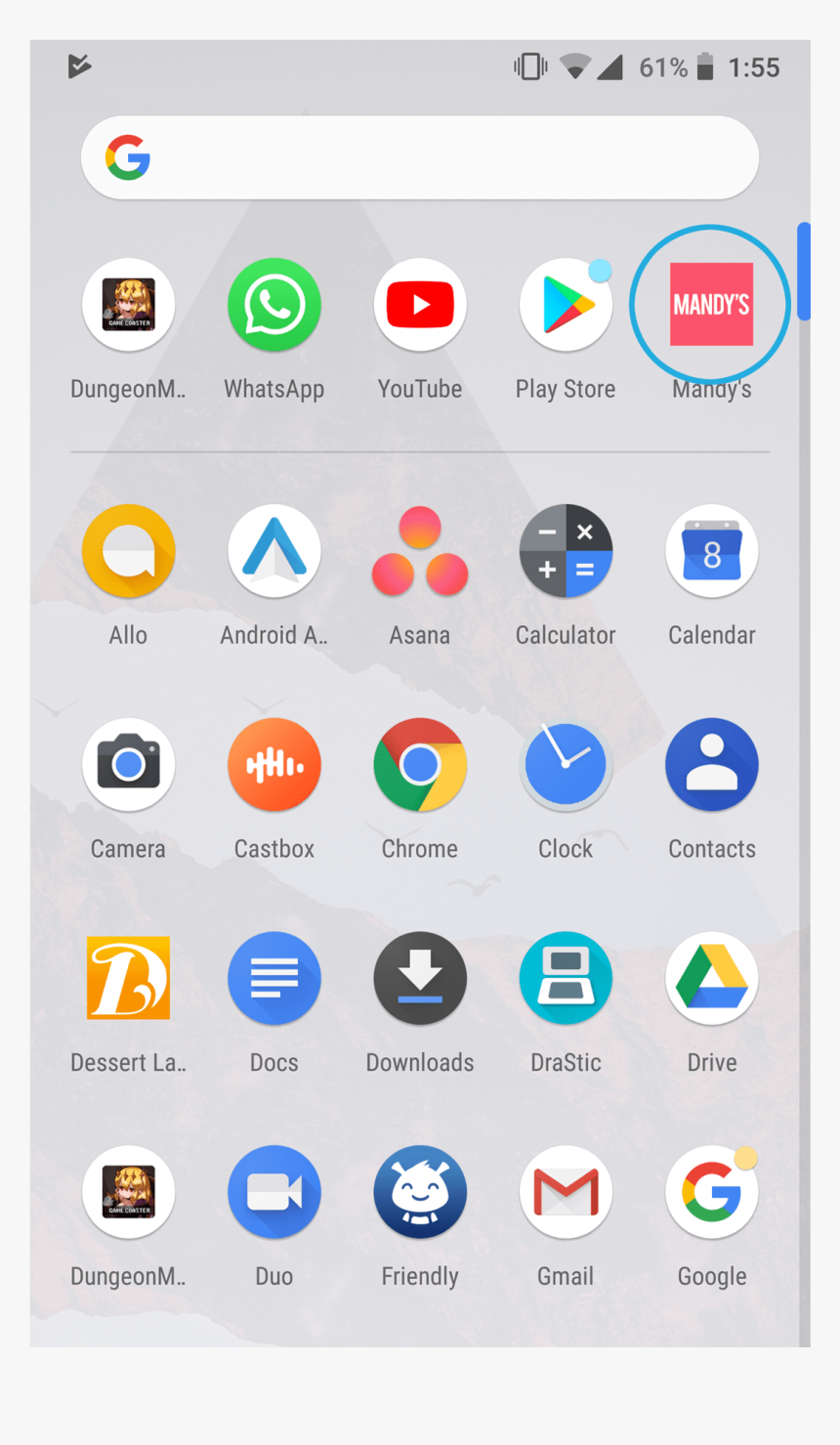In the image, we see a screenshot of an Android phone's home screen. In the top left corner, the notification bar shows that the Play Store app has been successfully downloaded, indicated by a corresponding icon. The visible apps on the screen include Dungeon Mobile, WhatsApp, YouTube, Play Store, and Mandis. Notably, the Mandis app is highlighted with a blue circle around it, with a blue scroll bar visible on the right side of the screen. The system time displayed on the device is 1:55, and the battery level stands at 61%. The WiFi signal strength appears to be low, while the network signal strength is full. Other visible apps on the screen include Camera, CastBox, Chrome, Clock, Contacts, Deserts, Land, Docs, and Downloads.